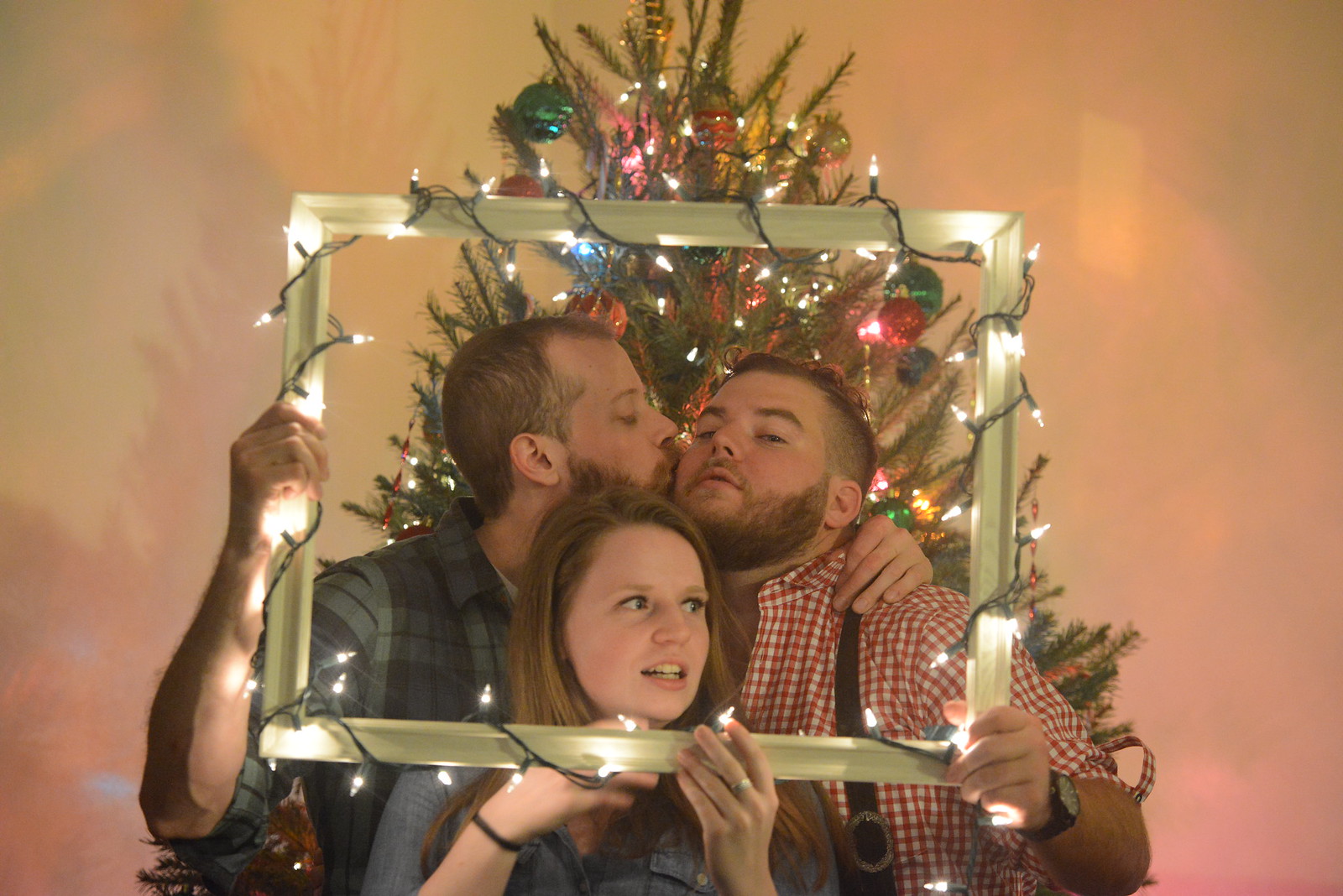The photograph captures a festive Christmas scene with three people posing in front of a green pine tree adorned with red and green ornaments and white Christmas lights. The backdrop has a peachy-purplish hue, adding a warm glow to the image. In the foreground, two men stand in the background holding a white or cream-colored frame wrapped in twinkling white Christmas lights. The man on the left, dressed in a blue plaid shirt, is affectionately kissing the man on the right, who is wearing a red and white checkered shirt. Positioned in front of the frame and looking off to the right of the photograph, is a woman whose left hand rests on the bottom of the illuminated frame. The overall ambiance is cheerful and festive, capturing the essence of a joyful Christmas celebration.